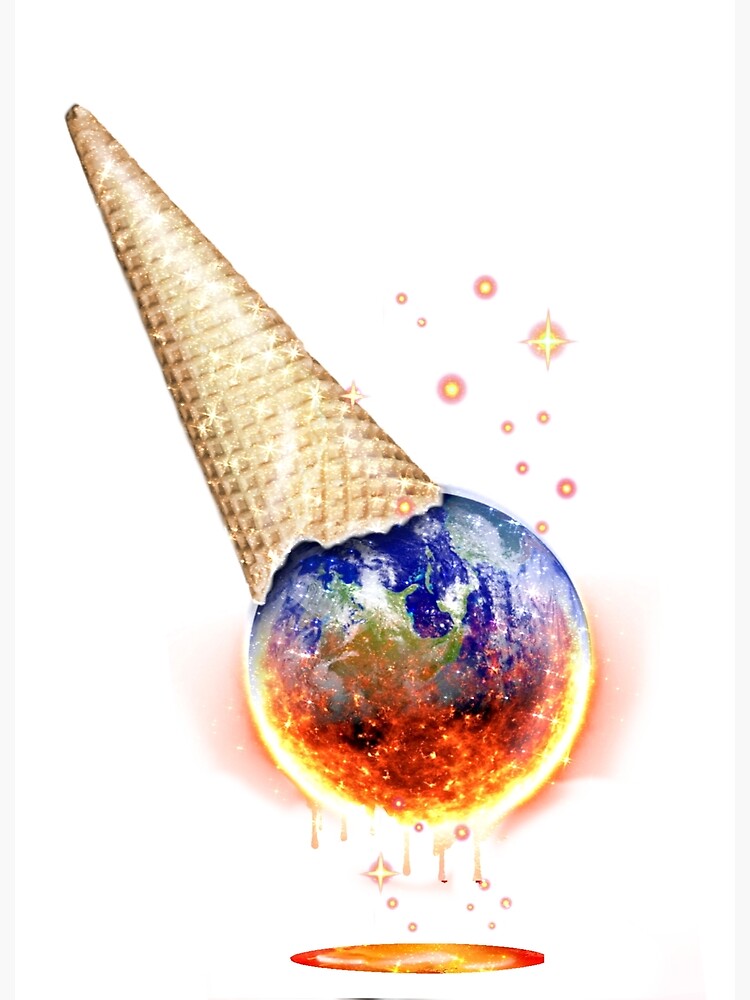This pixel art presents a striking depiction of the Earth as a melting ice cream cone. The cone, a tan-colored, stylized sugar cone with visible waffly ridges, is positioned diagonally with its point aiming up to the left, resembling the hour hand at 11 o'clock on a clock face. The Earth, illustrated as a scoop of ice cream, showcases prominent blue oceans and green continents, notably North America adorned with white clouds.

However, the lower half of the globe transforms dramatically, descending into a fiery portrayal. The serene blue gradually gives way to dark red, then to a luminous orange and yellow, mimicking molten lava as it drips from the Earth’s surface. These drips culminate in an orange, red, and yellow pool beneath the globe.

The backdrop is predominantly white, subtly shaded with a rosy hue around the globe. Above the Earth, various stylized stars, ranging from round to four-pointed, enhance the celestial theme. This artwork encapsulates a powerful visual metaphor, juxtaposing the ice cream cone's playful innocence with the alarming imagery of a planet under severe strain.